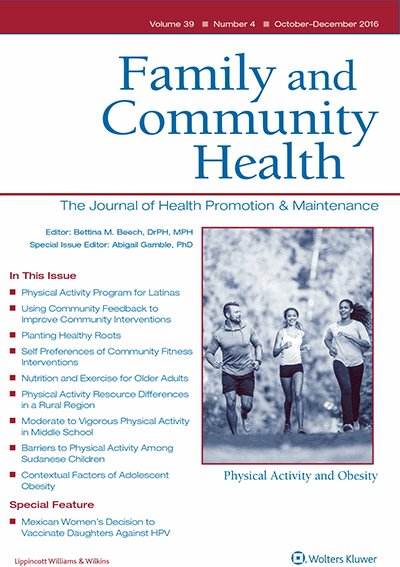The image showcases the cover of the journal "Family and Community Health: The Journal of Health Promotion and Maintenance." It is Volume 39, Number 4, from October to December 2016, published by Wolters Kluwer. The cover displays a red banner at the top with the journal's title prominently featured. The editors are listed as Bettina Beach, PhD, and special issue editor Abigail Gamble, PhD. The cover features an image on the lower right side of a white man and two Latina women jogging, with the caption "Physical Activity and Obesity." This issue covers a variety of topics, including a physical activity program for Latinas, using community feedback to improve interventions, planting healthy roots, self-preferences in community fitness, nutrition and exercise for older adults, differences in physical activity resources in rural areas, moderate to vigorous physical activity in middle schoolers, barriers to physical activity among Sudanese children, and contextual factors of adolescent obesity. A special feature focuses on Mexican women's decisions to vaccinate their daughters against HPV. The overall design emphasizes health and community wellness with a clean, mostly white background.